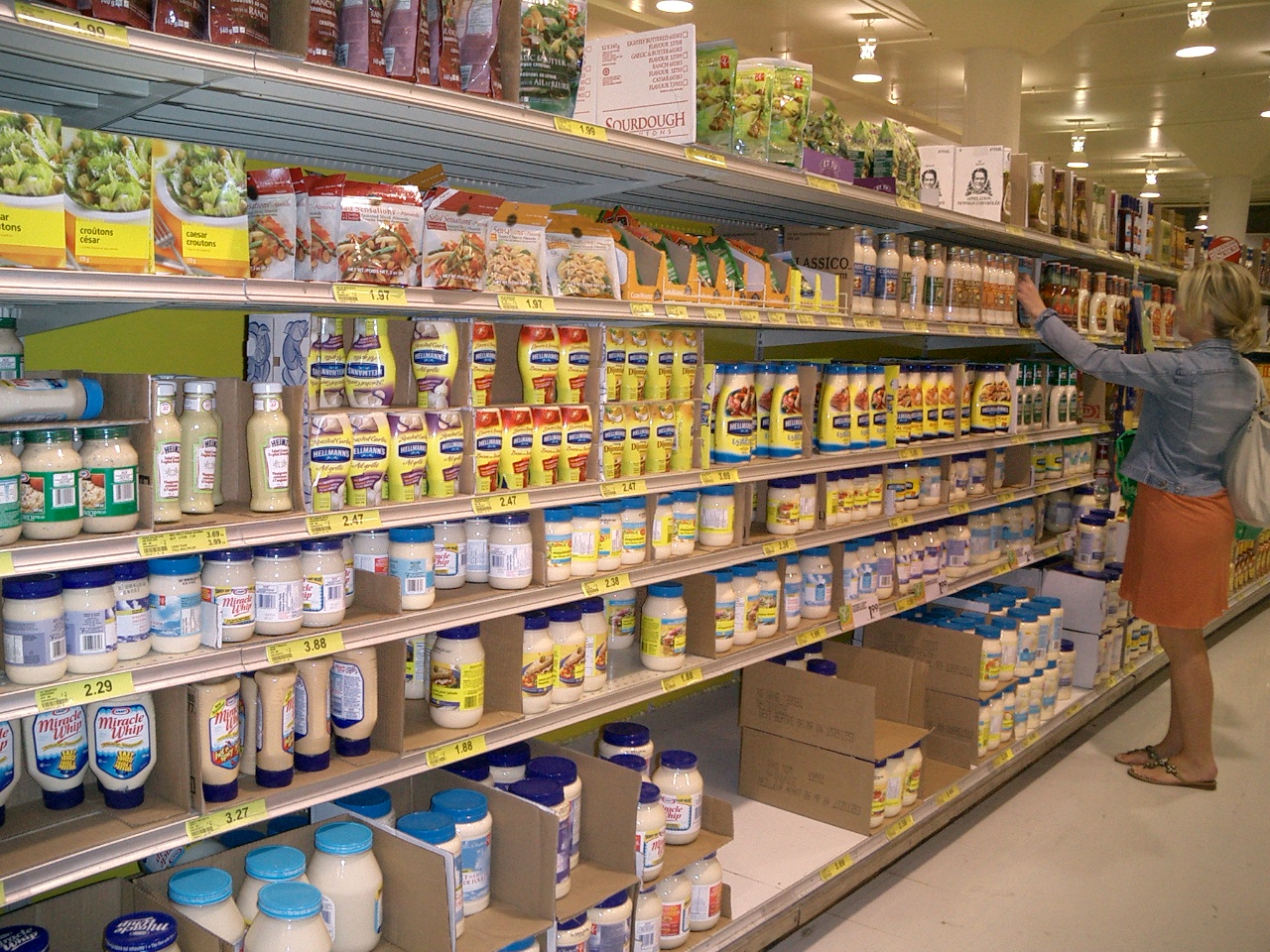The color photograph is a square shot of a grocery store aisle dedicated to mayonnaise and salad dressings. The aisle features six shelves, with the top part displaying bags of croutons. Below the croutons, various brands of salad dressings, including Paul Newman's, are visible, while the next three shelves down are filled with jars and pipes of mayonnaise. At the bottom, large containers of mayonnaise can be seen. Yellow price tags are visible underneath the products. The aisle is well-lit with circular ceiling lights set against a white, painted ceiling, giving the store a pleasant, inviting ambiance.

A woman is prominently featured in the image, positioned along the right side of the frame as she reaches for a product on one of the shelves. She has blonde hair and is wearing a jean jacket over an orange skirt or dress, paired with sandals. A gray purse is draped over her right shoulder.